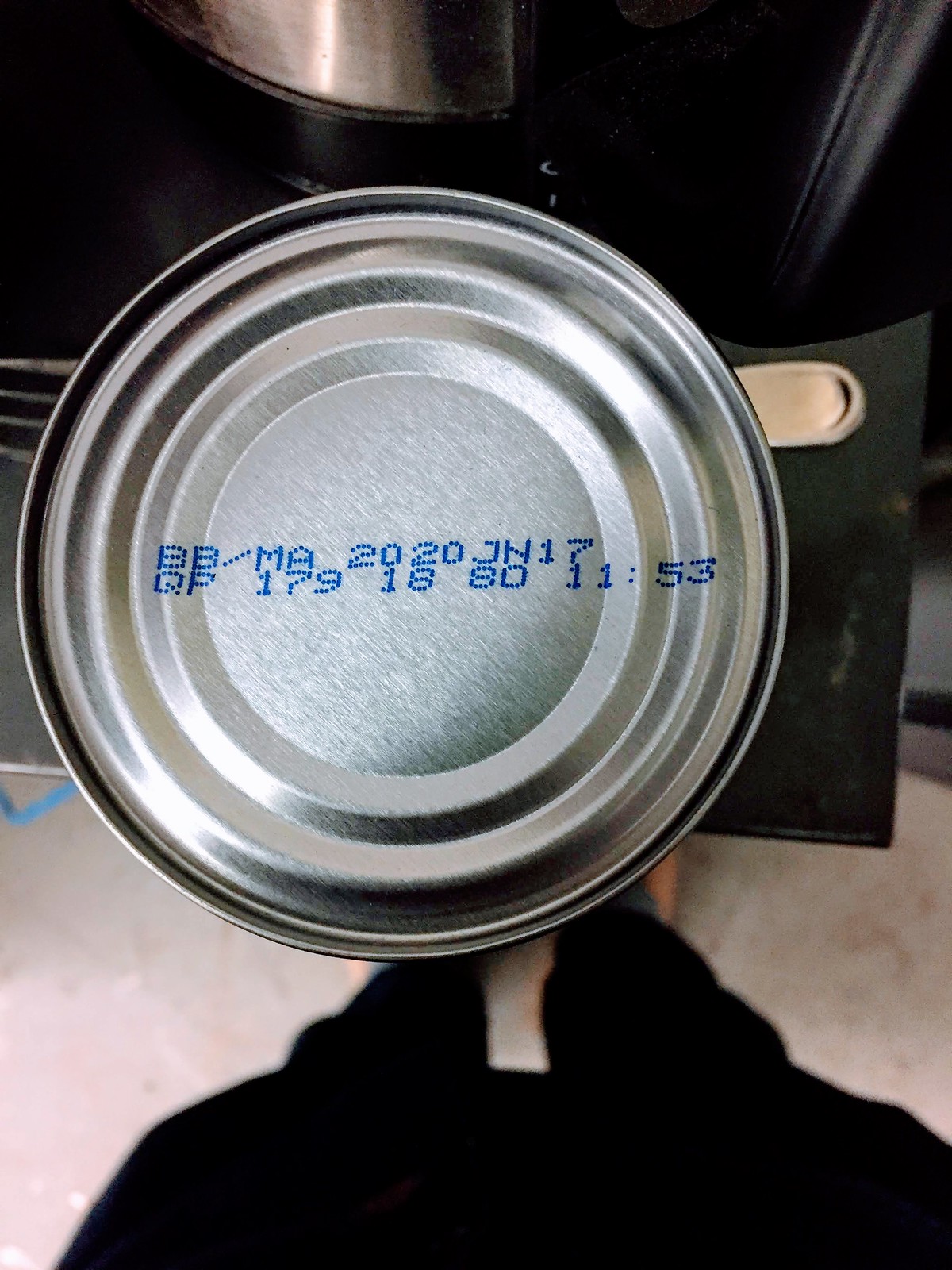This close-up photograph captures a scene in a kitchen viewed from above. At the center is a silver, cylindrical can of food resting on a black kitchen counter. The top of the unopened can features an expiration date and packaging information in dark blue text reading "BB/MA 2020 JN17" and "QP 179 18 80 11:53." Nearby, there's a small, indeterminate silver object. In the background, blurred yet noticeable, is a stainless steel and black plastic appliance that resembles a coffee maker. The person taking the photograph, dressed in black pants and a black shirt, is standing barefoot on a white floor with light brown splotches, possibly tile or linoleum, adding contrast to the sleek kitchen counter.